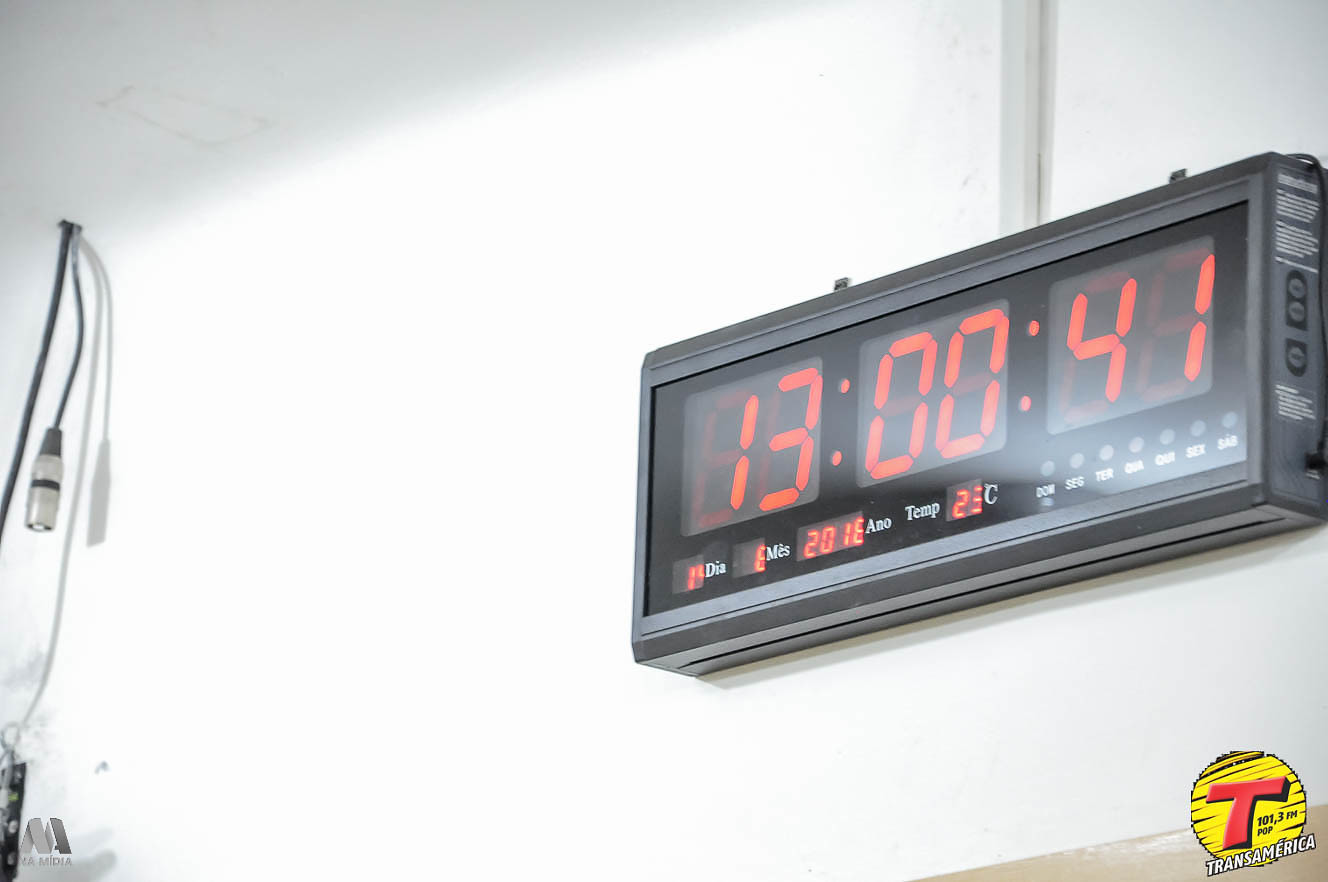The image depicts a highly detailed scene of a black, red-LED digital clock mounted on a white wall. The clock displays the numbers "13:00:41," suggesting it could be either 1:00 PM and 41 seconds or a countdown/elapsed time of 13 minutes and 41 seconds. Beneath the time, there is more text displaying "DIA", with the number 14, "MES", partly visible as either 8 or 6, "2016", and "AÑO". Additionally, the temperature is indicated as "23 degrees Celsius". Abbreviations for the days of the week, starting with "DCR" and including "TER", "SES", "SEX", and "SAD", are listed with dot markers above and below them. On the right side of the clock are white instructions and grey buttons with black borders for adjustments. The scene captures the clock mounted above a doorway, with a wire hanging down from the ceiling to the left of it. The photograph suggests a modern and digital setting, possibly from a video game or digital art piece, and shows no human presence. In the bottom right corner, there is a logo featuring a yellow circle with a red "T" labeled "103.3FM, POP, Transamerica".